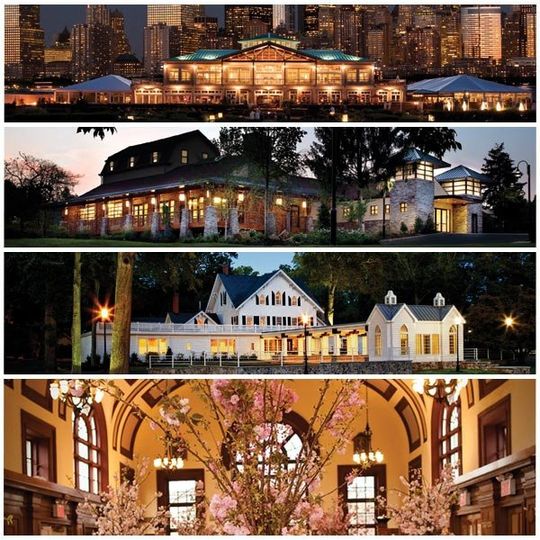This image collage, divided into four vertically stacked rectangular panels, showcases various elaborate structures and scenes, suggesting venues for grand events like weddings. The topmost image presents an ornately lit and grand two-story resort building with a pointed green roof, adorned with large archways and illuminated by numerous lights. A giant blue tent is visible on either side of the building. Behind it, the skyline of a vibrant city filled with illuminated skyscrapers and large buildings provides a stunning backdrop. The second panel features a rustic log cabin or stone building set amidst trees, characterized by white concrete pillars and a gray roof, giving it a quaint yet luxurious appearance. An array of lit windows adds a warm glow to the scene. The third panel depicts a massive white mansion with an elongated front area and a blue roof, situated in a similarly rustic setting with visible trees and open sky. The mansion’s extensive hallway and numerous lit-up features contribute to its grandiosity. The bottom panel transports the viewer inside a structure with a beautifully arched ceiling, where long-stemmed pink flowers, reminiscent of cherry blossoms, extend centrally, creating a picturesque and serene indoor corridor. The combined essence of this collage encapsulates a blend of opulence and natural beauty, ideal for sophisticated gatherings.